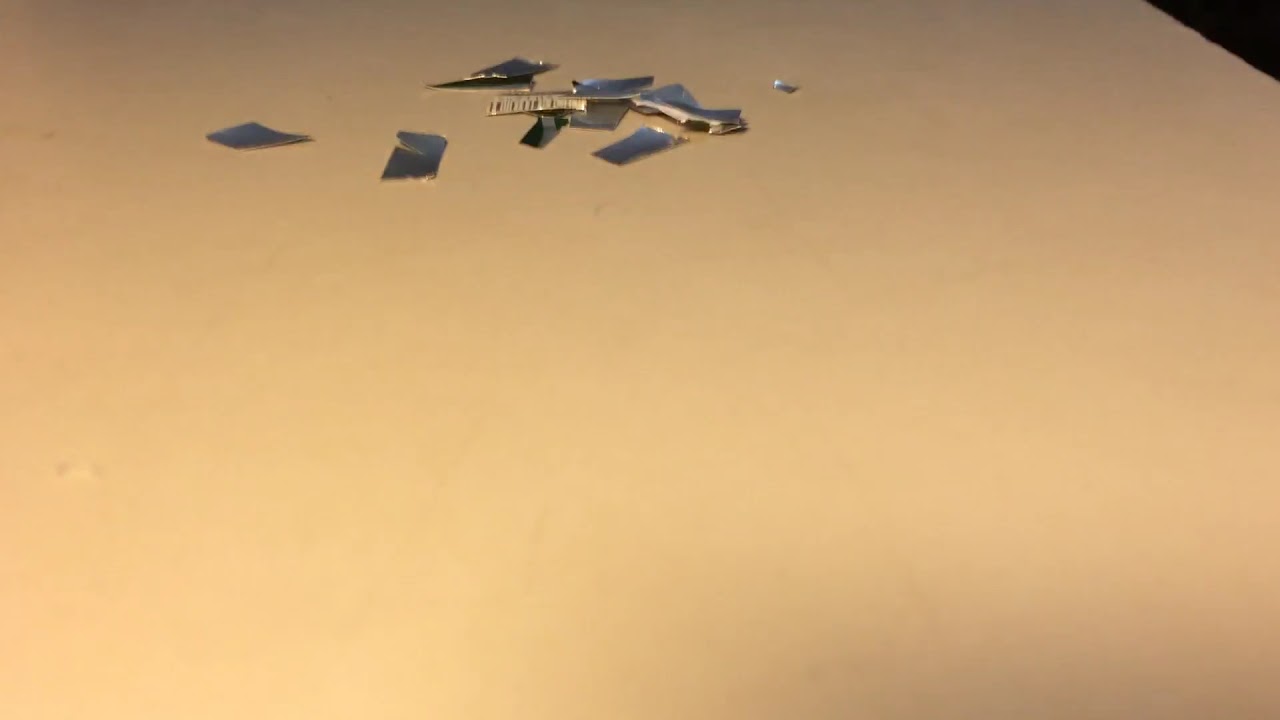The image features a plain, nondescript white or light tan surface that could be a tabletop or the top of a cupboard. The surface lacks any grain or texture, presenting a smooth, uninterrupted color. In the upper right corner, there's a small black triangle. Scattered across the upper middle section, slightly skewed to the left, are multiple small rectangular pieces of shiny, silver metal. The metal appears to be crudely cut, with some pieces showing bent edges while others have smoother finishes. These metallic pieces, varying in size but none particularly large, are both piled on top of and laid apart from each other. The exact thickness of the metal strips is indeterminate, though they give an impression of being relatively thin, possibly cut from aluminum foil or cans. The positioning and the reflective nature of the metal lend a scattered, almost chaotic look to the overall composition.